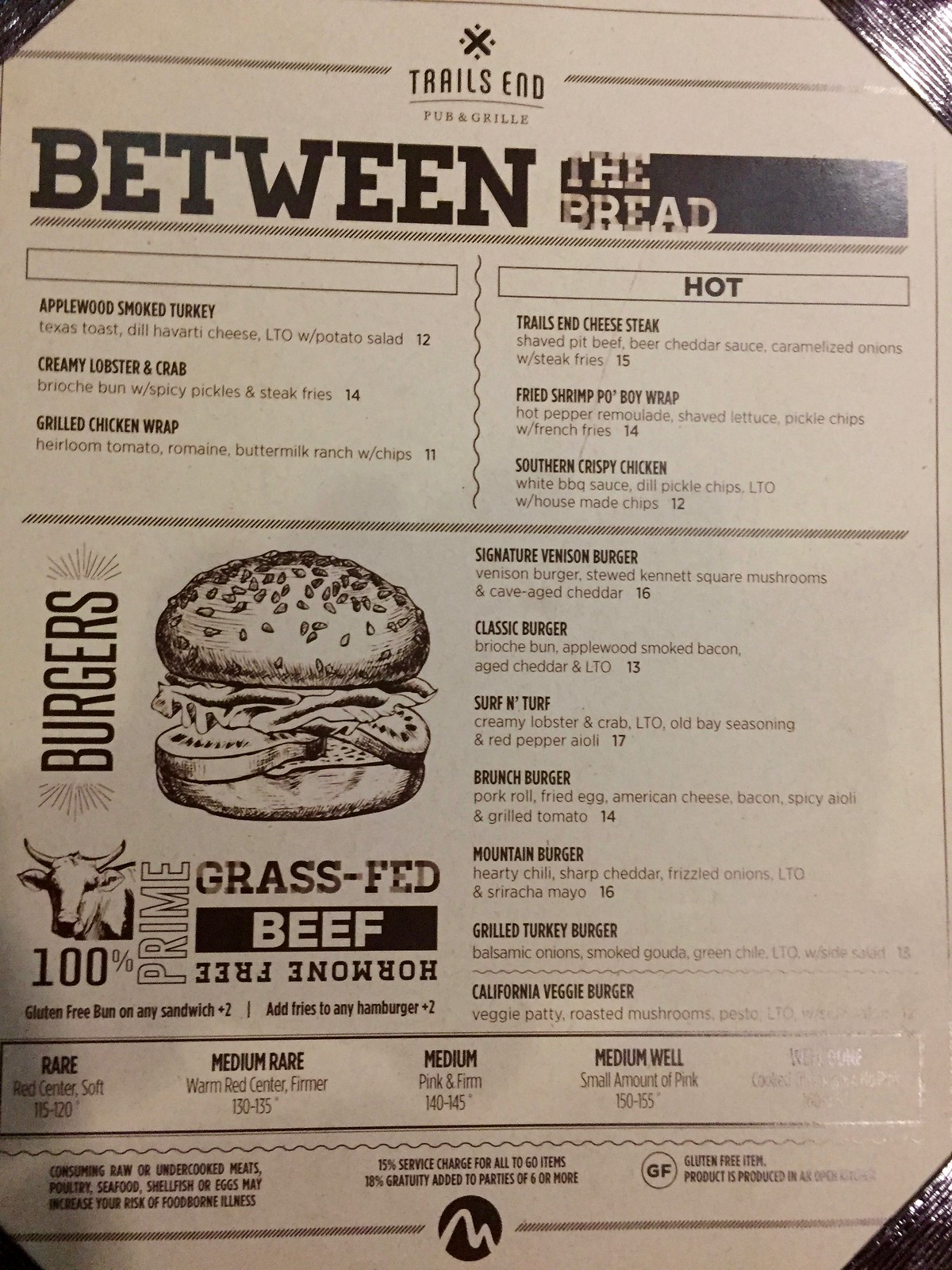The menu page from Trails End Pub and Grill is neatly presented in an off-white color with all-black font. It is secured in the corners with what appears to be angled, leather-like straps, giving it a classic, leather portfolio appearance. At the top of the page is the Trails End Pub and Grill logo, adding a touch of brand identity.

The title "Between the Bread" is prominently displayed at the top. Below this title, the menu is divided into sections. On the top left, there are sandwich options listed: Applewood Smoked Turkey, Creamy Lobster and Crab, and Grilled Chicken Wrap. To the right, in a section labeled "Hot," the offerings include Trails End Cheese Steak, Fried Shrimp Po'Boy Wrap, and Southern Crispy Chicken.

A dividing line separates these items from the burger section. Centrally located, a black and white image of a sesame seed bun hamburger is displayed. Next to this image, the word "Burgers" is written vertically. Underneath is a small cow's head emblem with the label "Prime, Grass-Fed Beef, Hormone-Free." Information about cooking temperatures and doneness levels is provided below this emblem, detailing Rare, Medium Rare, and other options.

To the right of the burger image, various burger options are listed along with their prices. These include: Signature Venison Burger, Classic Burger, Surf and Turf, Brunch Burger, Mountain Burger, Grilled Turkey Burger, and California Veggie Burger. This comprehensive listing caters to a variety of tastes and preferences, ensuring there's a choice for everyone.